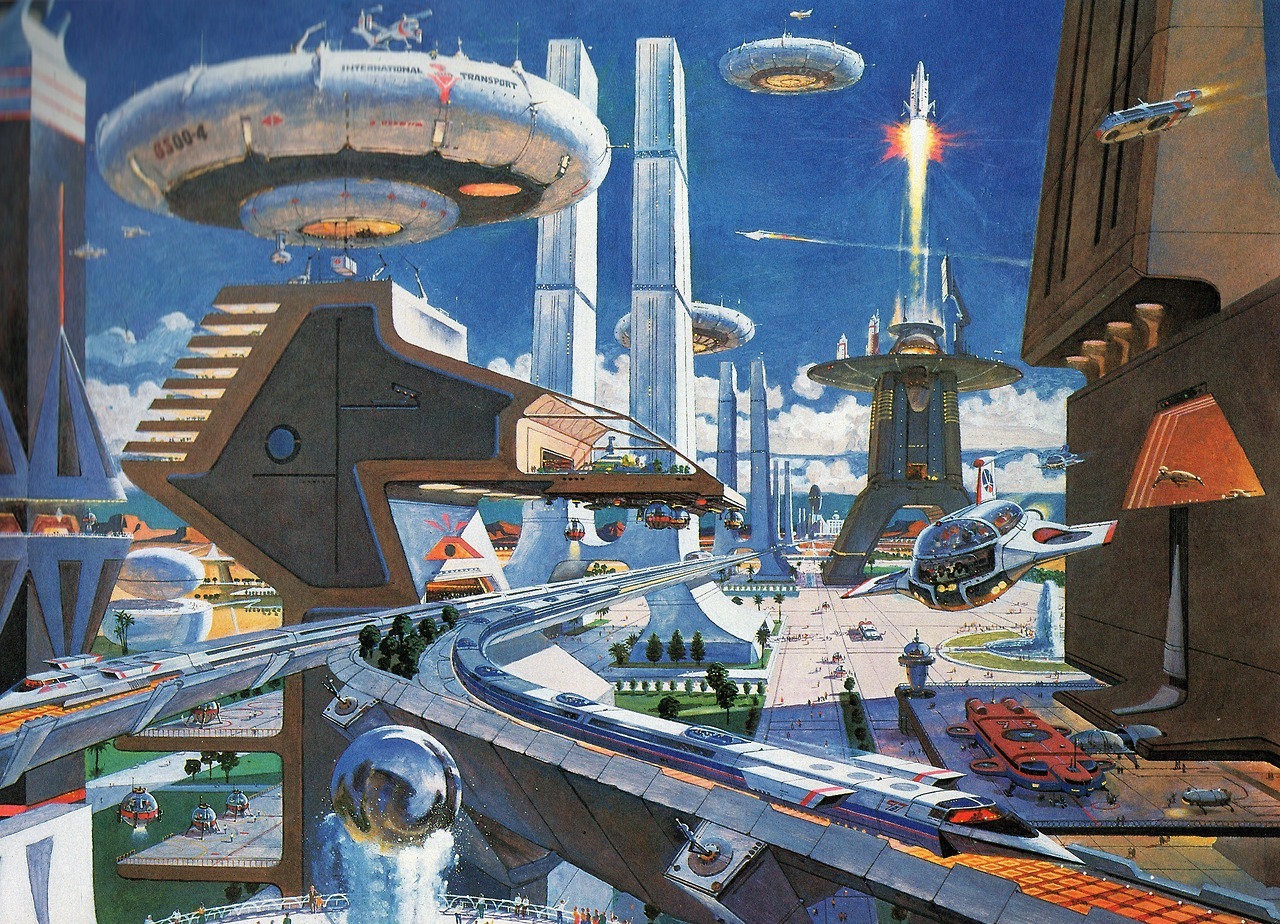This artwork is a highly detailed depiction of a futuristic metropolis, reminiscent of the cinematic and thematic visions seen in “The World of Tomorrow” and other utopian narratives. The cityscape is dominated by towering, slender buildings on both sides, creating a symmetrical balance. These buildings are arched and vast, suggesting advanced architectural innovations. Traversing the scene are multiple layers of sleek, aerodynamic trams, some featuring rocket or jet propulsion. These trams move dynamically from the lower right to the center, and then curve back towards the upper right, supported by massive columns that elevate them above the ground.

In the skies, a variety of flying vehicles fill the airspace, including hot rod-styled flying cars, hovering buses in both the left and right center, and numerous flying saucer-like spacecraft. Particularly notable are the hovering, cylindrical platforms that seem to serve as docking stations for these spacecraft. On the right side, rockets are prominently featured, with some launching from tall platforms. The background showcases a serene blue sky dotted with fluffy white clouds, offering a stark contrast to the bustling, yet orderly futuristic setting below. Sparse patches of grass and trees are visible, adding a touch of nature to this otherwise heavily urbanized cityscape.

Overall, this image paints an idyllic, non-violent vision of a 22nd-century utopia, complete with advanced transportation networks and innovative urban designs, making it a vivid representation of humanity's future aspirations.